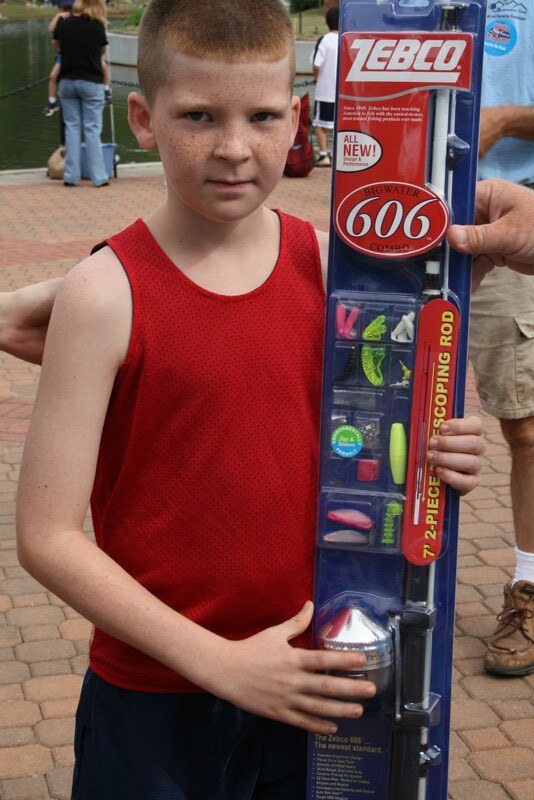In this vibrant, portrait-style photograph, we see a young boy, around seven or eight years old, with short red hair and freckles, wearing a red sleeveless shirt and blue pants. The boy is smiling at the camera, proudly holding up a Zebco Big Water 606 Combo, a seven-foot, two-piece telescoping fishing rod still in its packaging. The rod features a silver reel and comes with various accessories, including floats, all neatly arranged on a piece of plastic. The packaging prominently displays the brand name "Zebco" and the phrases "All New" and "Big Water 606." He is assisted by an adult hand visible on the right, which helps hold up the large package. Another adult, dressed in a light blue shirt and khaki shorts with boot-like shoes and white socks, stands in the background. The scene is set on a terracotta brick patio, with other out-of-focus individuals adding a sense of liveliness to this waterside backdrop.